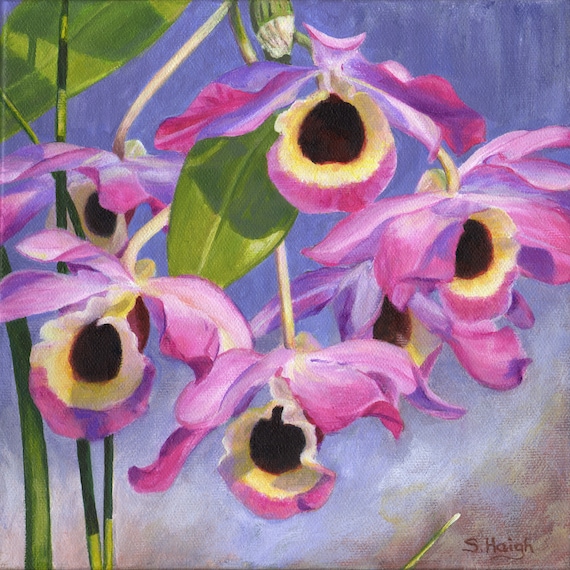This image depicts a photographic painting of orchid-like flowers with a detailed and vibrant composition. The main focal point is a cluster of flowers characterized by long green stalks that hang downwards. The petals are shades of purple and pink, with intricate detailing in their structure. Each flower boasts a brown-tubed center, encircled by a yellow halo, and culminating in purplish-pink tips. Surrounding the flowers are long, green leaves, and the image includes pods of unbloomed flowers in the background, adding depth to the scene.

The background starts as a light grayish-blue, gradually transitioning to a darker hue as it ascends. In the bottom right corner, there's an area of grayish-brown which frames the artist's signature, "S. Haigh." The overall style of the painting gives a slightly blurred, soft-focus effect, enhancing the delicate beauty of the flowers and their surroundings.